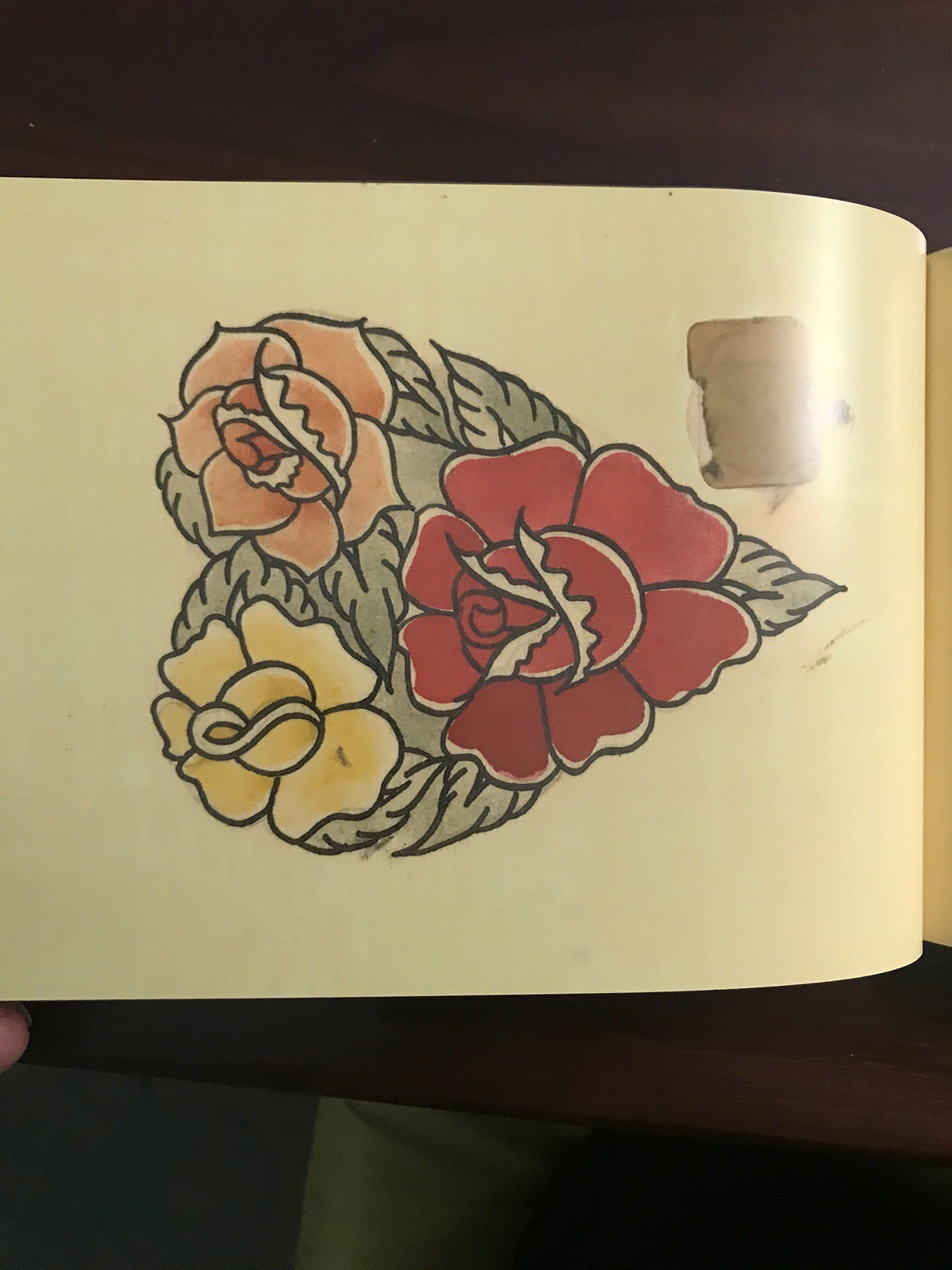A hand-drawn illustration depicts three roses arranged in the shape of a heart, with a vibrant yellow rose on the left side, an orange rose at the right peak, and a deep red rose at the bottom point. The intricate leaves of the roses create the heart-shaped background. The entire heart motif is rotated 90 degrees to the left, giving the impression of a sideways heart. The drawing, created with markers, is set against a white piece of paper. However, the photograph capturing this artwork was taken in a dim room without flash, causing the colors to appear faded.